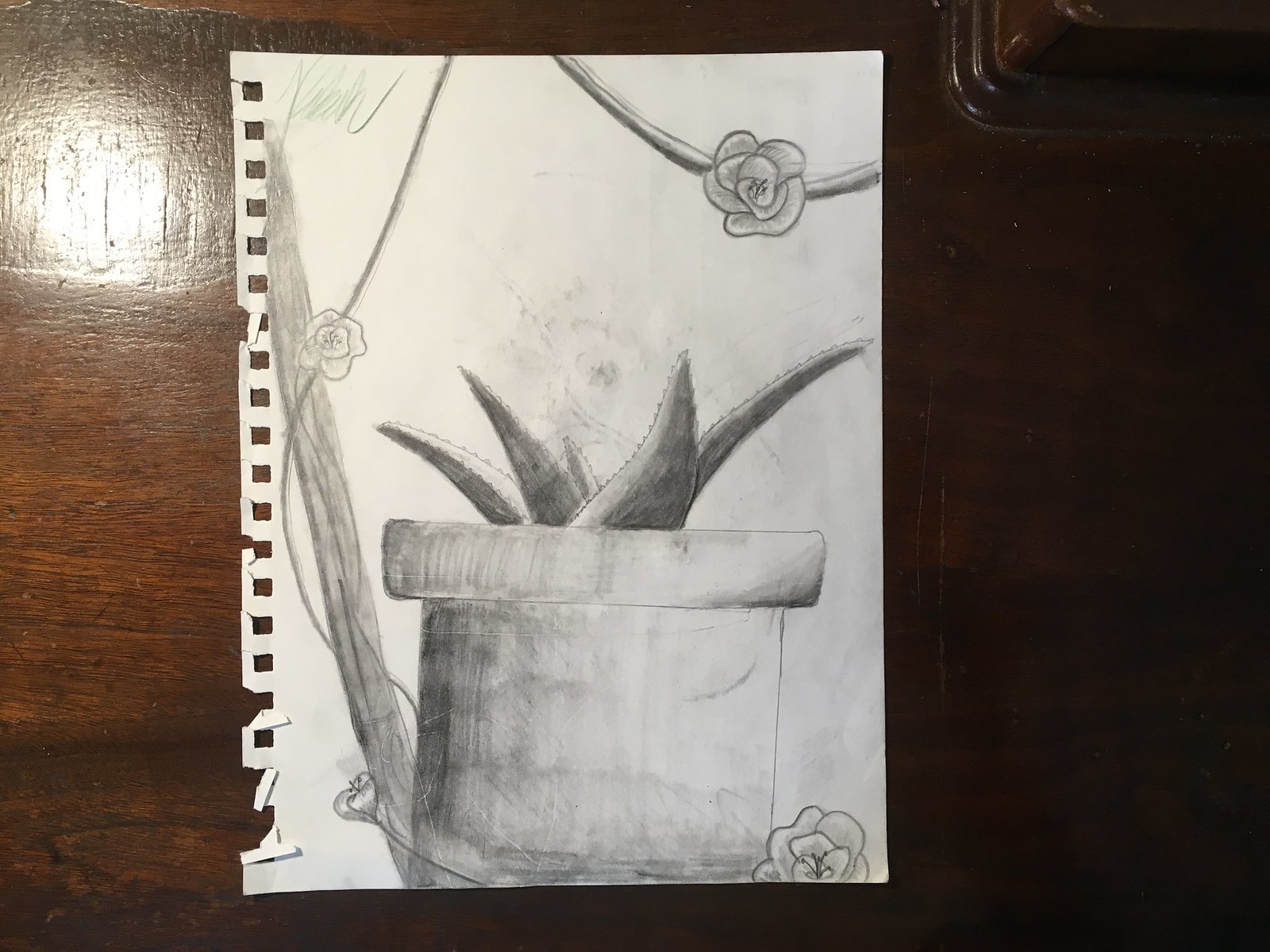A detailed sketch is rendered on a white sheet of paper, with rich shading emphasizing various elements. The focal point is a meticulously shaded flower pot, housing an aloe plant with five distinct, pointed leaves. The greenery is accompanied by intricately dotted flowers resembling roses. A brown stick-like object emerges from the left side of the pot, adding an organic touch to the composition. The artist has paid careful attention to shading in several areas, creating depth and dimension in the sketch. In the upper left corner, a scribbled signature marks the work. The paper, torn at the edges where it was ripped from a notebook, rests on a sleek black desk, providing a striking contrast to the artwork.